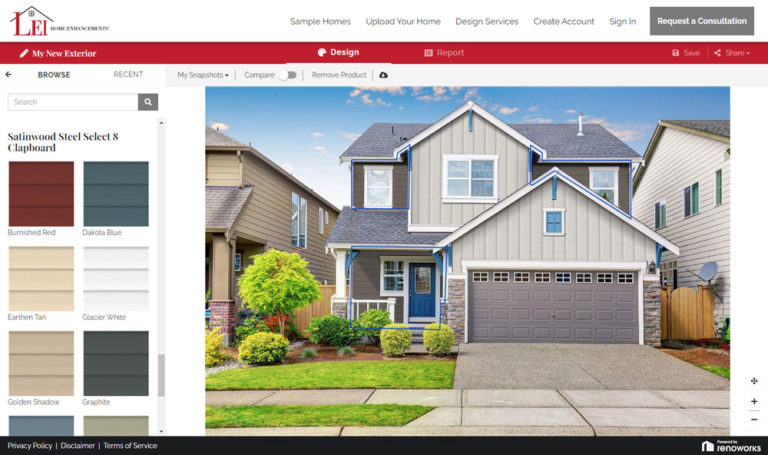This screenshot, taken from a website called LEI, showcases a painting company's digital interface. The image prominently features a house with various sections outlined in blue, indicating areas for potential color application. On the left side of the image, there are paint options listed: Satin Wood Steel Select Clapboard in multiple colors including Burnished Red, Dakota Blue, Earthen Tan, Glacier White, Golden Shadow, and Graphite. The house itself is presented in a combination of light gray and dark gray hues, with its front door painted a striking bright blue. The surrounding driveway and sidewalk are plain concrete, and the house is complemented by a well-maintained, small yet manicured front yard. Additional color options are mentioned below the visible colors but are not shown in the screenshot.